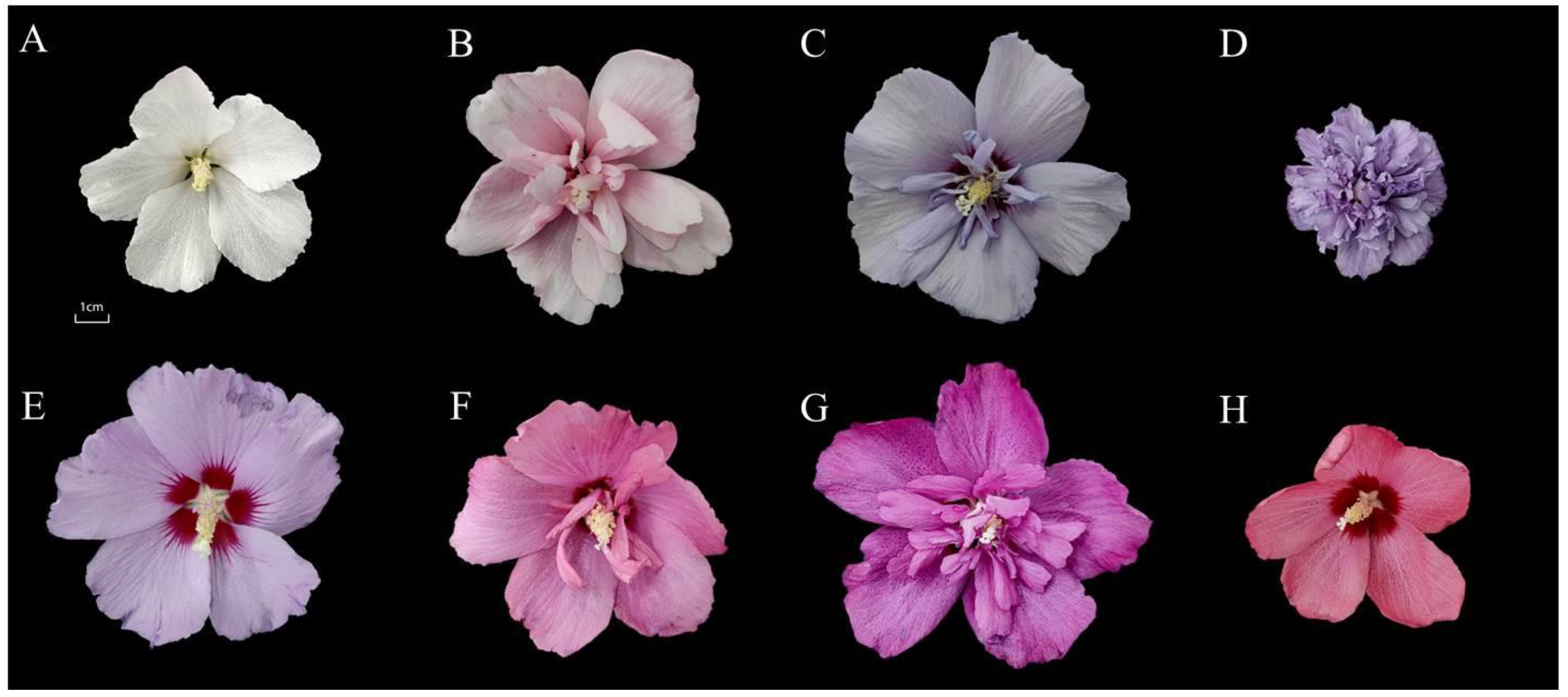The photograph features a collection of diverse flowers, arranged into two rows against a solid black background. Each flower in the top row is labeled with a white letter in the upper left corner, from A to D, while those in the bottom row are labeled E to H—all in Times New Roman font. The top row includes: A, a white flower with five petals and small white blossom stems; B, a light pink bloom with five large outer petals and smaller ones in the center; C, a light lavender flower with five outer petals and smaller central ones; and D, a tightly bunched purple carnation. The bottom row consists of: E, a light lavender flower with a reddish base to its petals; F, a bold pink flower; G, a vibrant magenta flower; and H, a rosy orange-red flower. There is also a 1cm scale mark placed under the first flower in the bottom row, emphasizing the size of these delicate blooms.